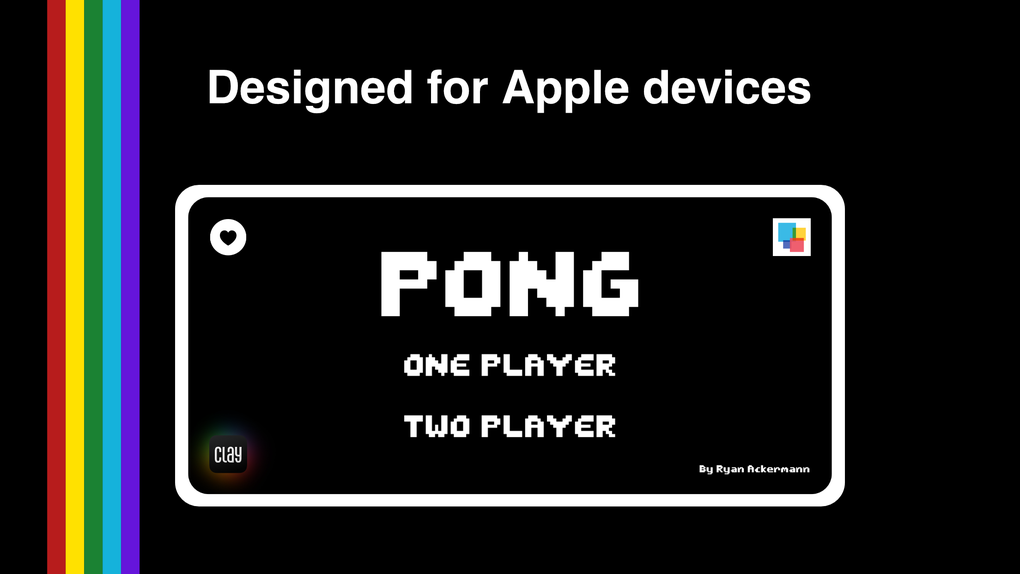The advertisement for the classic video game Pong features a sleek black background. To the left, vertical stripes in vibrant red, yellow, green, blue, and purple add a splash of color. At the top of the poster, white text reads "Designed for Apple devices." Central to the image is a horizontally oriented iPhone-like device with a white border, displaying "Pong" with the options for 1 player or 2 player on a black screen. The top left corner of this device shows a heart icon inside a white circle, while the top right corner features four multicolored boxes. In smaller text at the bottom right, the name "Buy Ryan Ackerman" suggests the creator or promoter of the game. The bottom left corner features the logo for Klay, potentially another company involved in the game's revival. The design emphasizes the availability of the nostalgic game Pong on Apple devices, blending classic arcade aesthetics with modern technology.